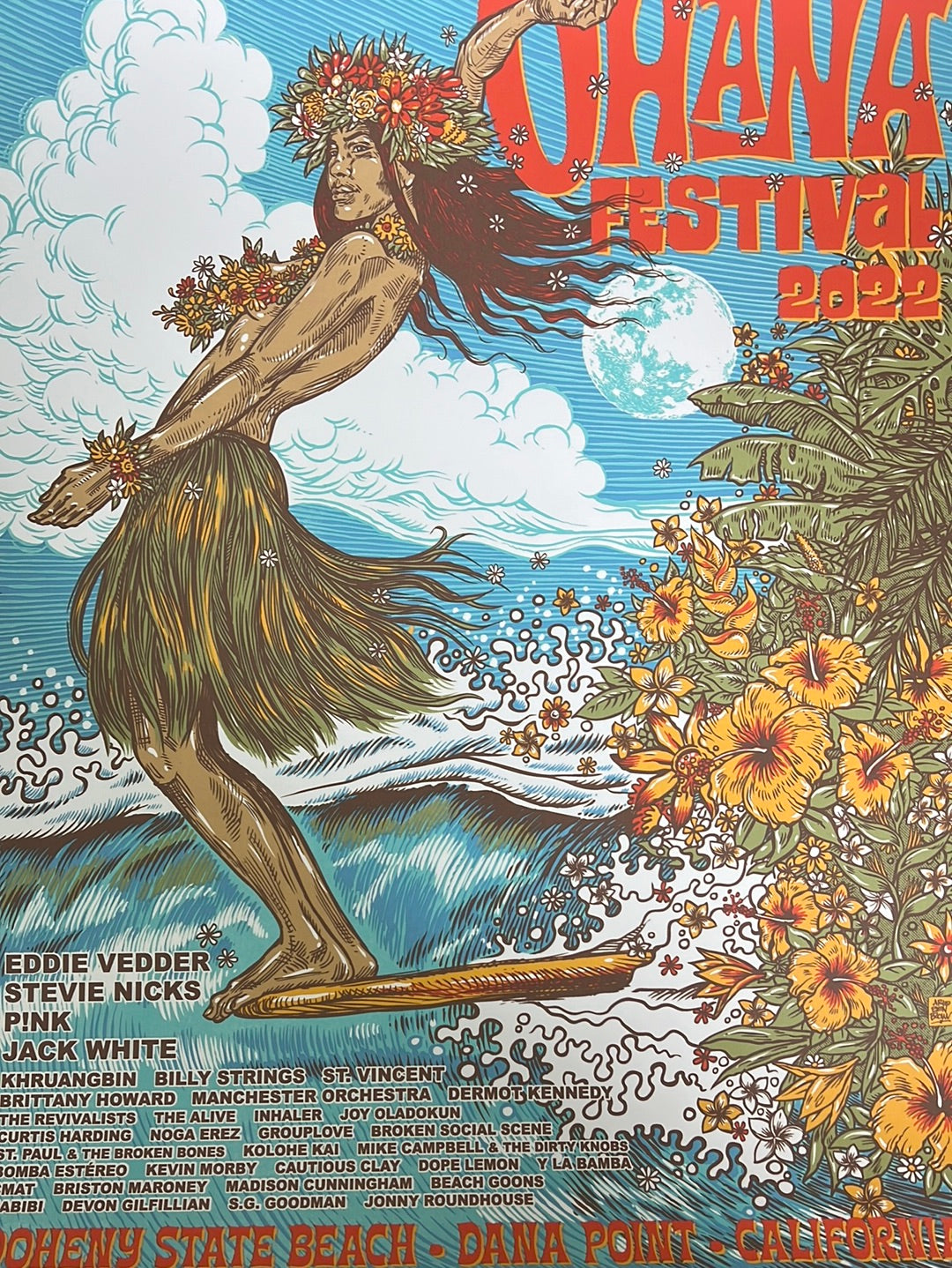This vibrant poster is for the Ohana Festival 2022. It features a captivating comic-style illustration of a Hawaiian woman surfing on ocean waves. The backdrop is a vivid blue sky with white clouds and a large moon overhead. The surfer is adorned with flowers in her long, flowing hair, a floral headdress, and floral wristbands. She is topless with strategically placed flowers covering her breasts and wears a traditional hula grass skirt. To her right, there are yellow flowers and lush Hawaiian plants. The festival's name, "Ohana Festival 2022," is prominently displayed in red letters with an orange outline in the top right corner. The bottom left corner lists the headliners Eddie Vedder, Stevie Nicks, Pink, and Jack White, along with dozens of other musical acts in black text. Below this, the location is given as Doheny State Beach, Dana Point, California. The image, busy and colorful, captures the essence of a tropical paradise and sets an energetic and festive tone.